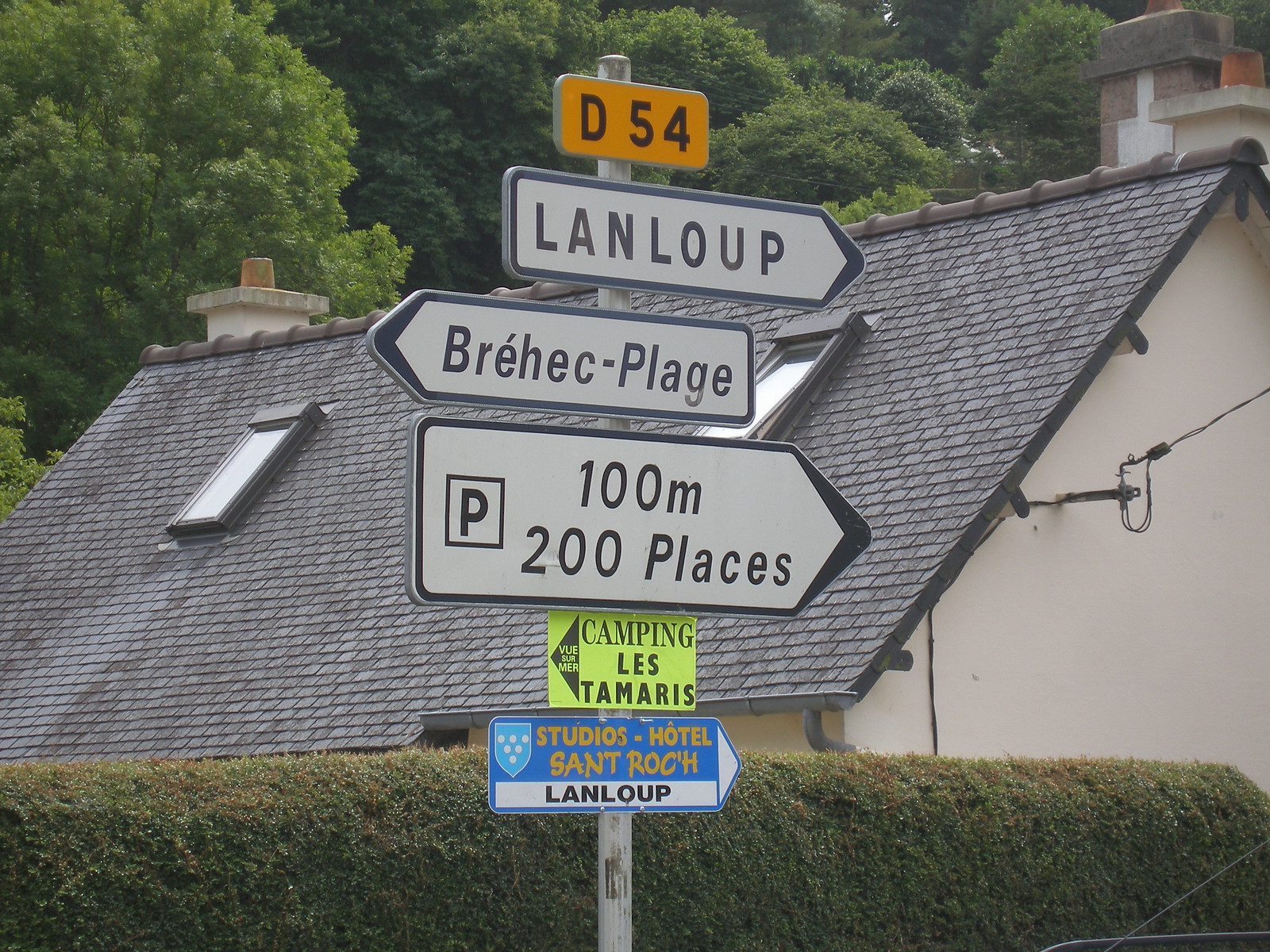This photograph captures a detailed street signpost on the side of an unseen road, covered in several directional and informational signs stacked vertically on a black and white pole. The topmost sign is a small yellow rectangle with black text reading "D54." Beneath it, the next sign is white, labeled "Len Laupp," followed by another white sign reading "Brehek Plek." A larger white sign below directs towards a parking area, with text stating "100 meter, 200 places" accompanied by a parking symbol. Further down, a small yellow poster advertises "Camping Les Tamaris." The lowest sign, blue and white, mentions "Studios Hotel Saint Roach Len Laupp." 

In the background, a house with a tan stucco exterior and a gray, triangular roof complete with an open skylight and chimney is partly visible. The house is bordered by green-leaved trees. Some of the signs point in different directions, indicating various travel routes. Directly behind the signpost, there's a long hedge, contributing to the picturesque outdoor scene.